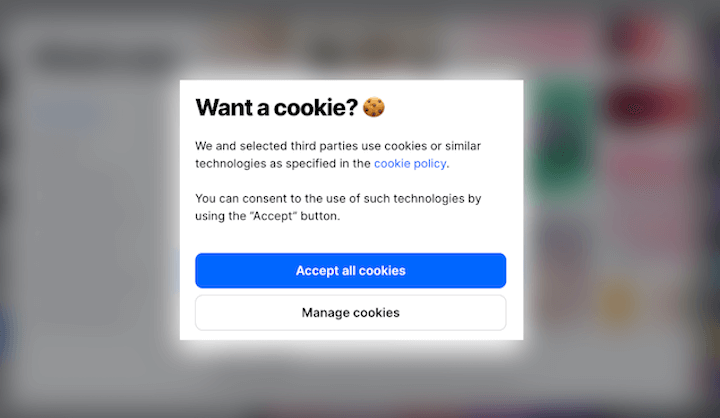The image features a very blurred, multi-colored box displaying vivid hues of pink, green, red, yellow, and purple. Central to this box is a pop-up notification with large black letters that read, "Want a cookie?" Accompanying the text is an image of a cookie, seemingly chocolate chip, dotted with small dark spots. 

Beneath this attention-grabbing header, the text states: "We and selected third parties use cookies or similar technologies as specified in the cookie policy." The phrase "cookie policy" is highlighted in blue, indicating it is a clickable link for more information.

Below this statement is a prominent button labeled "Accept" in quotation marks, and beside it, another button that says "Accept All Cookies" in blue font with curved edges. Underneath these buttons, there's a smaller white box with the option "Manage Cookies" written in black lettering, offering further customization for cookie preferences.

The background of the image is intentionally blurred, obscuring some information in the upper left-hand corner, hinting at a website containing various types of content highlighted in different colors. The specific details of the company or website remain indistinguishable due to the blurriness.